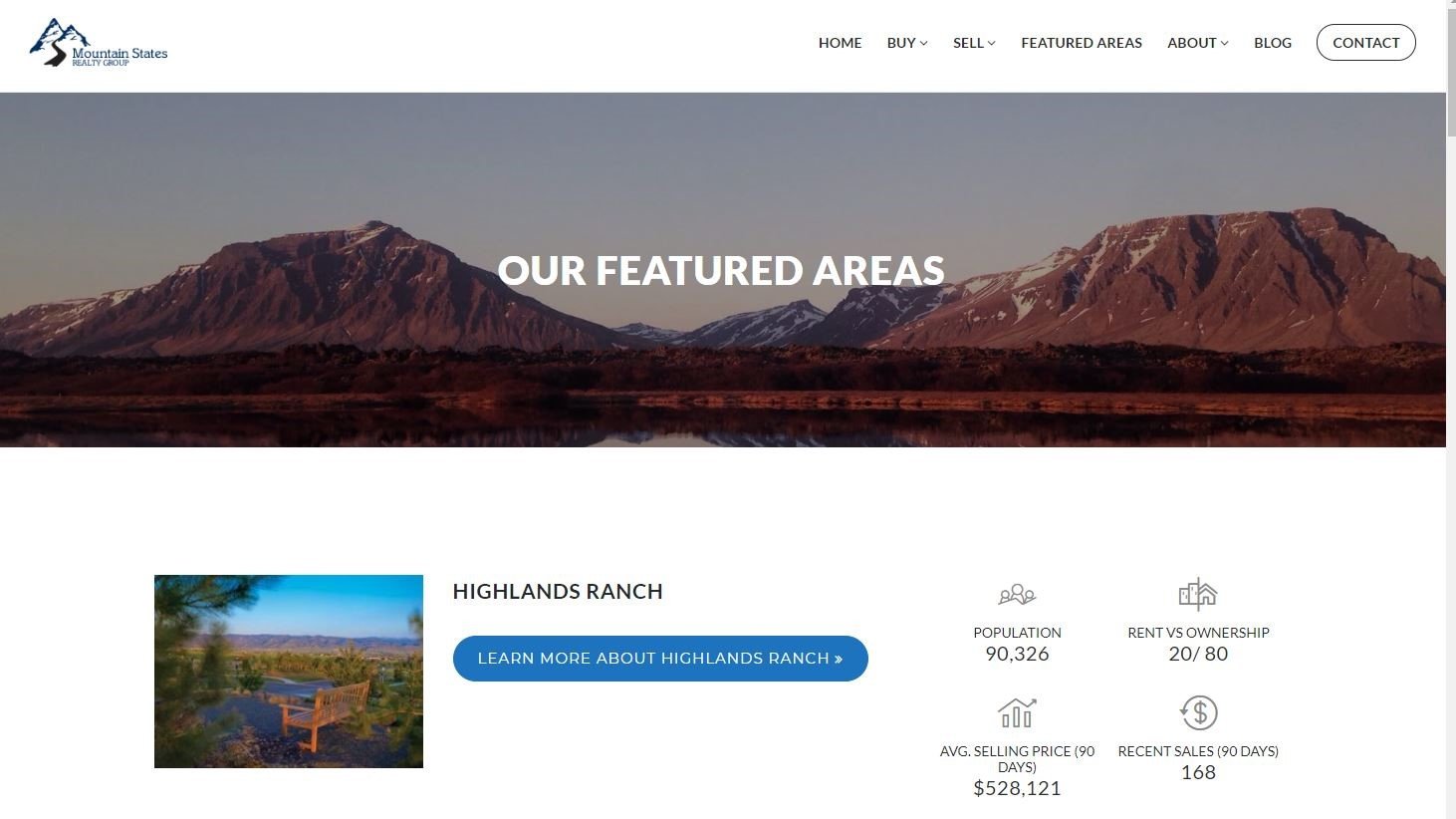The advertising website for the organization called Mountain States prominently displays its logo in the upper left-hand corner. The logo features two mountains with a river flowing out from between them, accompanied by the words "Mountain States" in small blue font. On the right-hand side of the top-line menu, visitors can find various drop-down features available on the site.

Dominating the width of the website, a large rectangular image showcases a breathtaking view of the lower foothills of the Rocky Mountains, characterized by their tall and brown-colored peaks. The image is labeled with the phrase "OUR FEATURED AREA" in bold, white, all-capital font.

Directly below the featured image, the website presents several options and information about the highlighted areas. Among these is the featured ranch called Highlands Ranch, accompanied by a small thumbnail photo. The section provides details about the ranch and related real estate sales, offering visitors an insightful glimpse into this particular area.